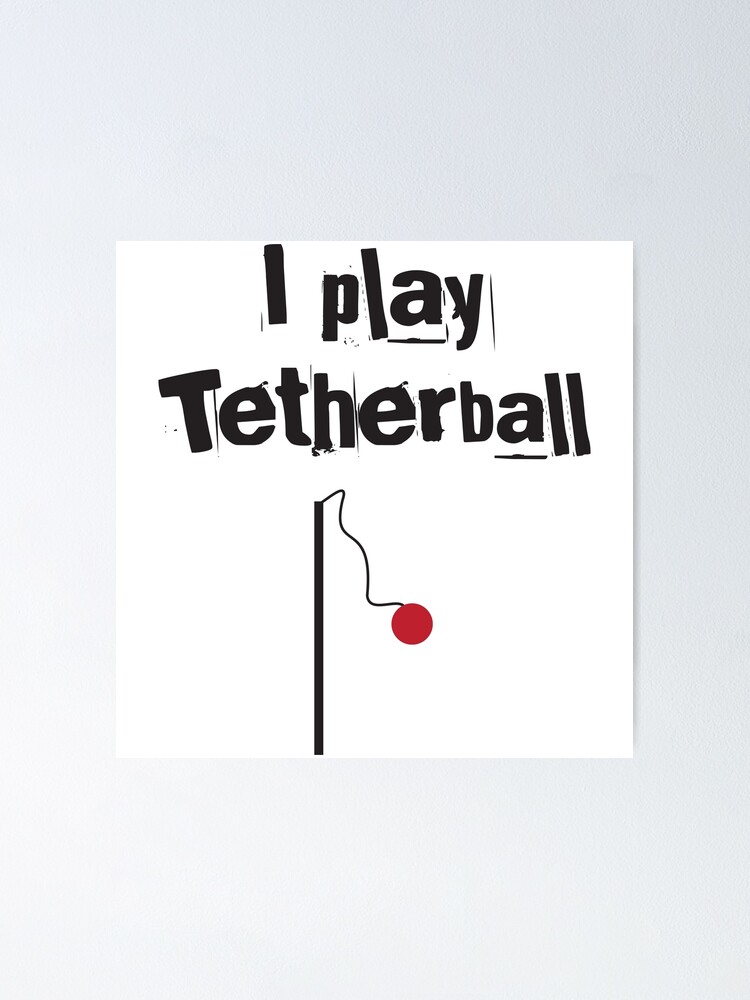This image features a tetherball game depicted on a white piece of paper, bordered by a blue frame which is about twice the width of the inner white section. Dominating the scene is a slender black pole that extends from the bottom and reaches halfway up the white paper. A black, zigzagging string hangs from the pole, with a bright red tetherball seemingly in motion at the end of the string. Above this illustration, bold black letters spell out "I play" at the top, and below that, the word "tetherball" is centered, with each "A" in the text underscored by a small line. The lettering appears rough and somewhat speckled, as though cut from a magazine or printed with slight imperfections. The plain white background accentuates the simplicity and childlike quality of the artwork.